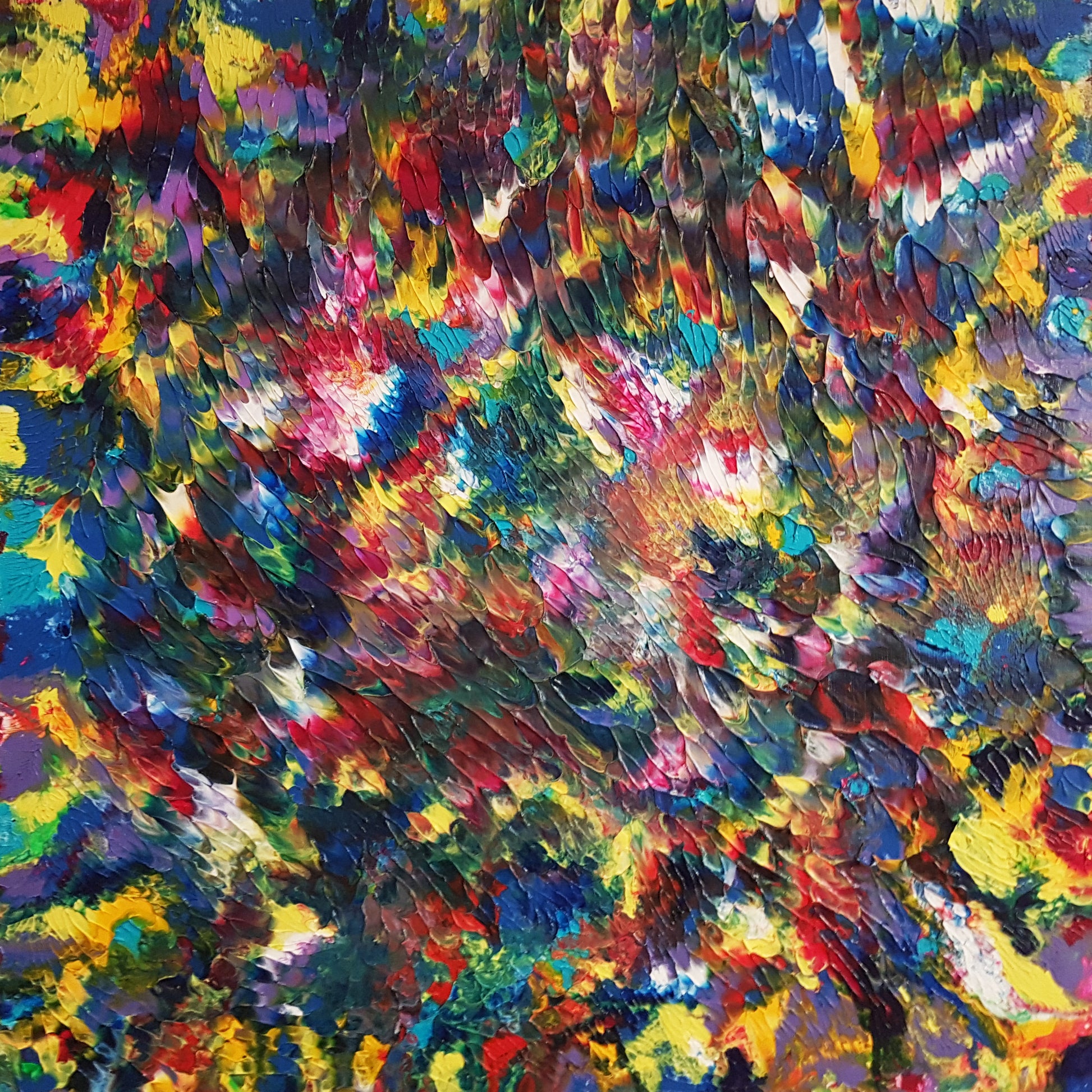This image is a vibrant, abstract painting characterized by a chaotic explosion of multi-colored brush strokes and splatters. The canvas is a visual cornucopia, featuring practically every hue imaginable - vivid reds, deep blues, lush greens, sunny yellows, soft pinks, occasional whites, and a few bold blacks. The painting lacks a defined structure, with colors seemingly randomly chosen and applied with varying pressure, but there is some discernible pattern in the brushwork. Vertical strokes dominate the top part of the painting, while in the middle, many strokes take a diagonal turn towards the bottom right. The overall effect is reminiscent of colorful seaweed growth or fish swimming freely, with globular splotches adding to the sensory overload. The dynamic colors and forms create a blurry, mesmerizing effect, compelling the viewer's eyes to roam and explore every inch of the canvas.